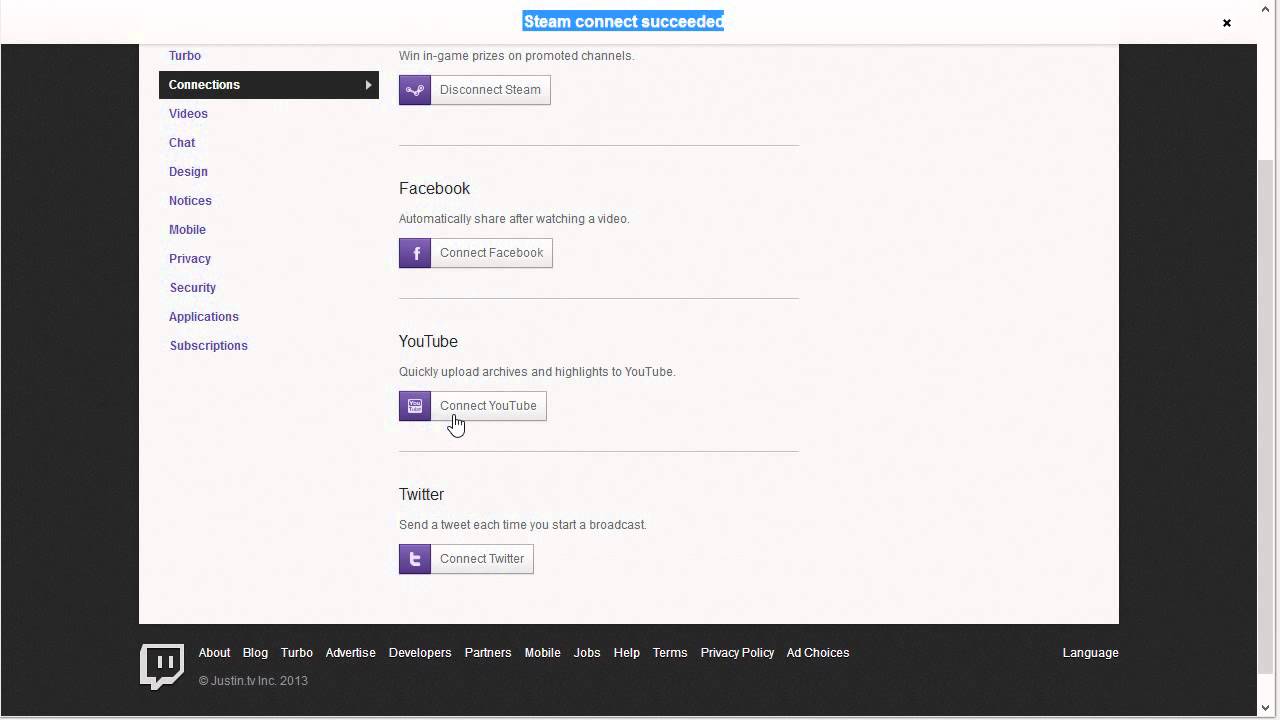The image is a screen capture from a website, showcasing various connection options and account settings. At the top of the image, there is a thin white bar, and a blue-highlighted notification that reads “Steam Connect succeeded."

Prominently displayed in the center against a black background is a large white pop-up box. On the left side of this box are clickable blue links labeled "Turbo" and "Connections." Inside the "Connections" section, written in white font on a black background, are various categories including Videos, Chat, Design, Notices, Mobile, Privacy, Security, Applications, and Subscriptions.

On the right side of the pop-up box, there are sections in black font alongside purple and gray clickable shortcuts. These shortcuts include "win in-game prizes on promoted channels," "Disconnect Steam," "Facebook: automatically share after watching a video" with a "Connect Facebook" button, "YouTube: quickly upload archives and highlights to YouTube" with a "Connect YouTube" button, and "Twitter: send a tweet each time you start a broadcast" accompanied by a "Connect to Twitter" button. A white cursor is visible hovering over the "Connect YouTube" button.

At the bottom of the page, additional options appear in white font, including About, Blog, Turbo, Advertise, Developers, Partners, Mobile Jobs, Help, Terms, Privacy, Policy, Ad Choices, Language, and a notice that reads “© Just Flynn LV Inc 2013.” No other notable elements are present in the image.